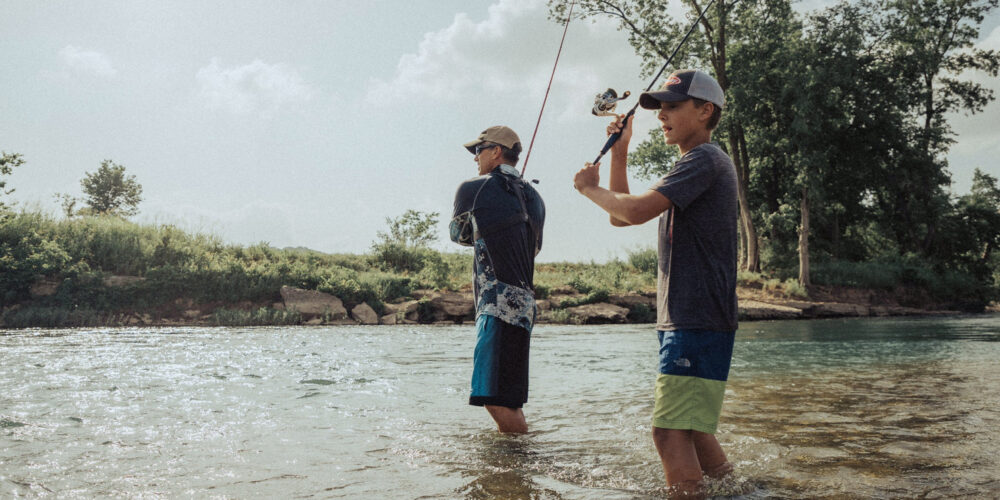In a scenic outdoor setting on a partly cloudy day, the photograph captures two young men, possibly teenagers, engaged in fly fishing while standing in ankle-deep, greenish-brown water. The young man in the foreground, who looks to be slightly younger, is wearing a black and white cap, a gray t-shirt, and blue and green swim trunks. He holds his fishing rod with both hands, poised to cast. Slightly behind him stands another young man wearing sunglasses, a tan cap, a dark shirt, and black and blue shorts. He has his fishing rod pulled back over his shoulder, ready to cast into the water. The background features a rocky bank leading to a grassy hill on the left, with a few trees visible to the right, all under a blue sky dotted with clouds.